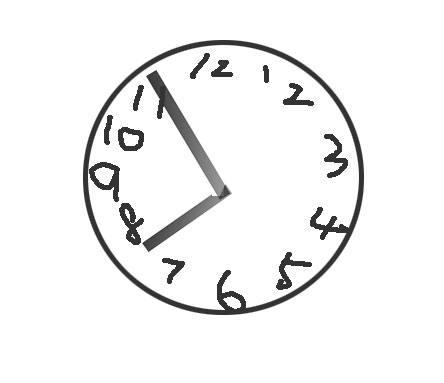The image captures a meticulously drawn perfect circle, within which resides a small, hand-numbered clock face. Each hour from 1 to 12 is scruffily placed, with some numerals appearing disproportionately larger or smaller than others. The digits, though legible, display a charmingly chaotic alignment. At the center, or rather where the center should be, two rectangular clock hands are affixed haphazardly. One is markedly wider than the other, and they converge slightly off-center, pointing towards approximately 7:55. The overall impression is one of endearing disorder—a clock that, despite its eccentricities and asymmetrical elements, undeniably functions as intended.